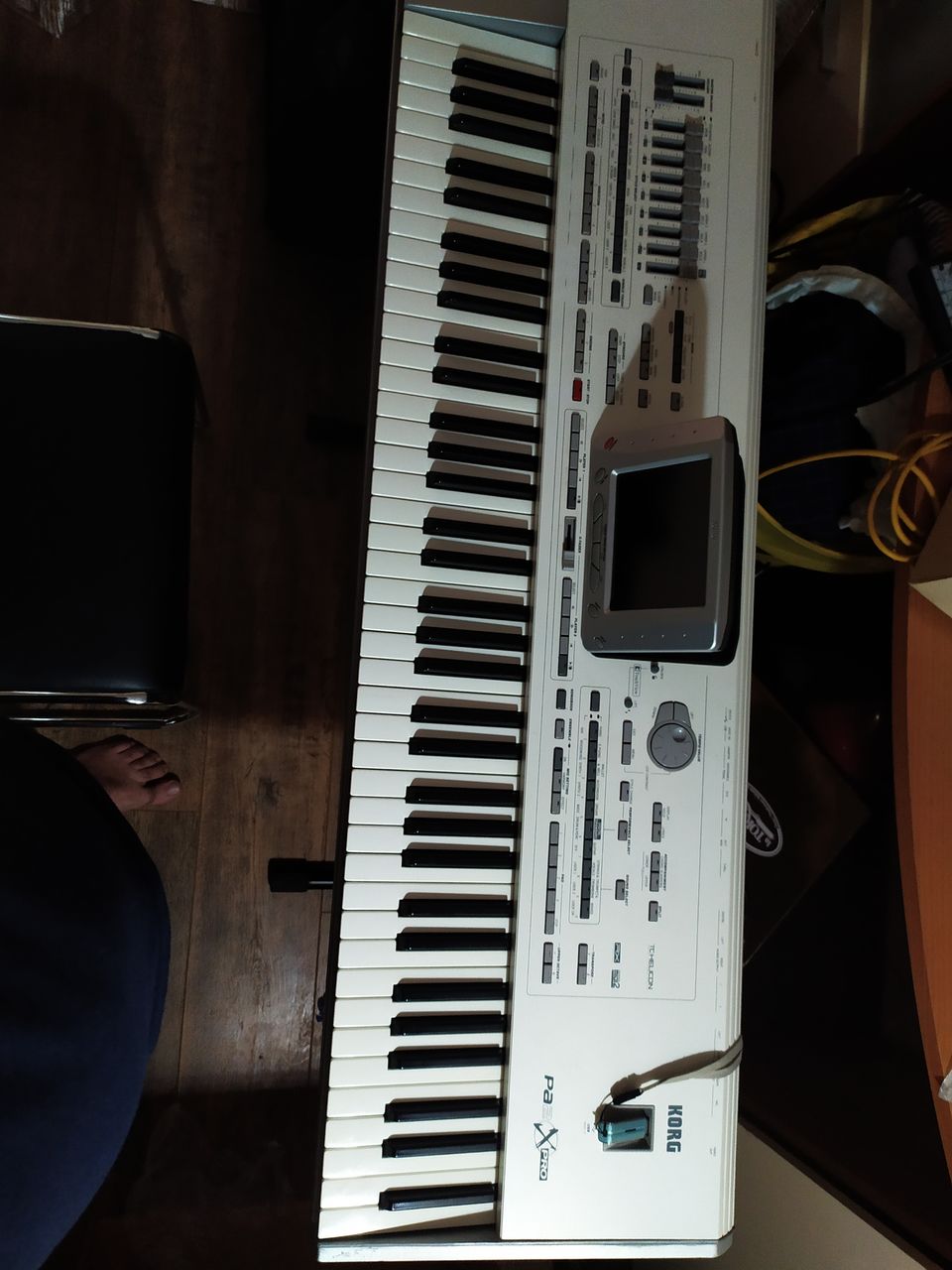The image showcases a sophisticated Korg electronic keyboard displayed in a vertical position. Central to the keyboard is a computer readout, although the screen is currently off, indicating the keyboard is not powered on. The power button, distinguishable by its green hue, is a prominent feature among an array of control options that include numerous sliding scales, a twist dial, and assorted buttons. This intricate instrument rests on a metal folding stand, characterized by its X-shaped design for stability. Adjacent to the stand is a small seat, presumably meant for the keyboard player. Partially visible in the frame is the player's left leg and foot, positioned on what appears to be a wooden or vinyl plank floor. The background details remain ambiguous, but there might be speakers situated behind the keyboard. Overall, the impressive and potentially costly keyboard setup suggests that the owner likely has considerable skill in playing the instrument.